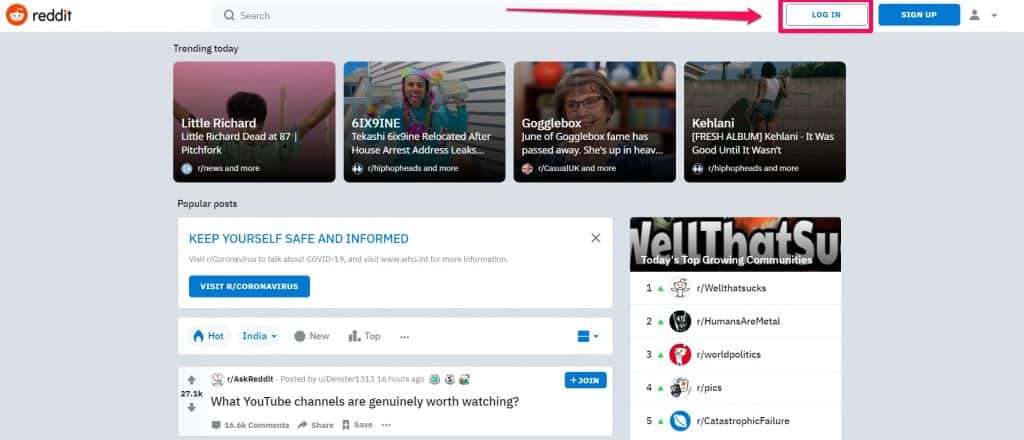This image appears to be a screenshot taken from Reddit. In the upper left-hand corner, the familiar Reddit logo and label are prominently displayed. Central to the image is a light blue search bar, emphasizing the platform's search functionality. A striking red arrow points from this search bar towards the login section, indicating the path for user login, which is shaded in blue and outlined in red.

To the right of the login section, there is a blue "Sign Up" button situated next to a generic profile icon. Below this, a heading reads "Trending Today," showcasing popular content. 

- The first trend features a small box with a picture of Little Richard accompanied by the text "6x9."
- Adjacent to this is an image of a girl adorned in blue, pink, and yellow attire.
- Following that is a mention of "Google Box" or "Goggle Box," paired with a photo of a short-haired woman wearing glasses.
- The last trend in this section highlights "Kehlani," with what appears to be a beach scene, although the details are dark and somewhat indistinct.

Beneath the "Trending Today" section, notable posts are highlighted under the “Popular Posts” heading:

- A prominent white box bears the message, "Keep Yourself Safe and Informed," instructing users to visit a certain link, although the exact URL is too small to decipher. This message is contained within a blue box.
- Another white box below it displays the text “Hot India New Top,” with another blue box to the end.
- Further down, a question reads, "What YouTube Channels Are Genuinely Worth Watching," again concluded with a blue box.

Towards the bottom of the screenshot, there's a caption stating, “Well, That's Sue,” accompanied by more images from Reddit. However, these images are very tiny and difficult to interpret.